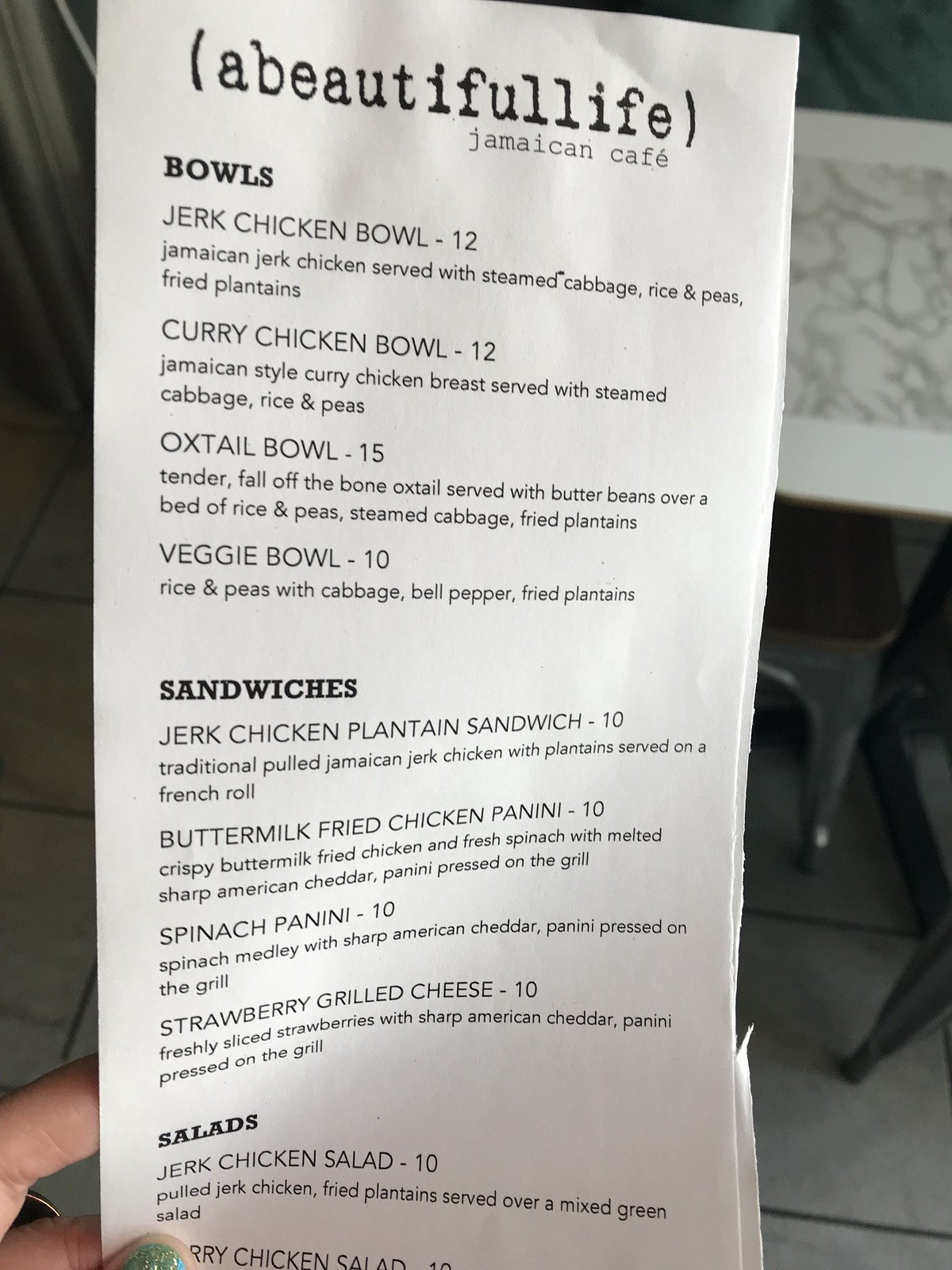A person is reading a menu at a restaurant called "a beautiful life (a beautiful full life)" photographed in portrait orientation. At the top right of the image, part of a table with a white border and faux marbled inset is visible, along with chair legs that appear to be wide, tapering metal with wooden seats. The floor, glimpsed along the left side and bottom right corner of the photo, features light-colored tiles with dark grout.

In the bottom left corner, a woman's hand with glittery silver nail polish on her thumb and visible parts of her index and middle fingers is holding the back of the menu, which is a slim, long, narrow, disposable paper menu.

The restaurant name "a beautiful life (a beautiful full life)" is printed in bold, lowercase typewriter-style font. Below it, "Jamaican cafe" is written in lowercase. The menu lists different categories of food, each with the item name in all capitals, followed by a description in lowercase and the price with a hyphen and the number, omitting the dollar sign. 

Items under the "Bowls" section include:
- JERK CHICKEN BOWL - 12: Jamaican jerk chicken served with steamed cabbage, rice and peas, and fried plantains.
- CURRY CHICKEN BOWL - 12: Jamaican style curry chicken breast served with steamed cabbage, rice and peas.
- OXTAIL BOWL - 15: Tender fall-off-the-bone oxtail served with butter beans over a bed of rice and peas, with steamed cabbage and fried plantains.
- VEGGIE BOWL - 10: Rice and peas with cabbage, bell pepper, and fried plantains.

Under the "Sandwiches" section:
- JERK CHICKEN PLANTAIN SANDWICH - 10.
- BUTTERMILK FRIED CHICKEN PANINI - 10.
- SPINACH PANINI - 10.
- STRAWBERRY GRILLED CHEESE - 10.

Finally, under "Salads," there are:
- JERK CHICKEN SALAD - 10.
- CURRY CHICKEN SALAD - 10.

The image shows that the menu continues below, but it is cropped off at the bottom.